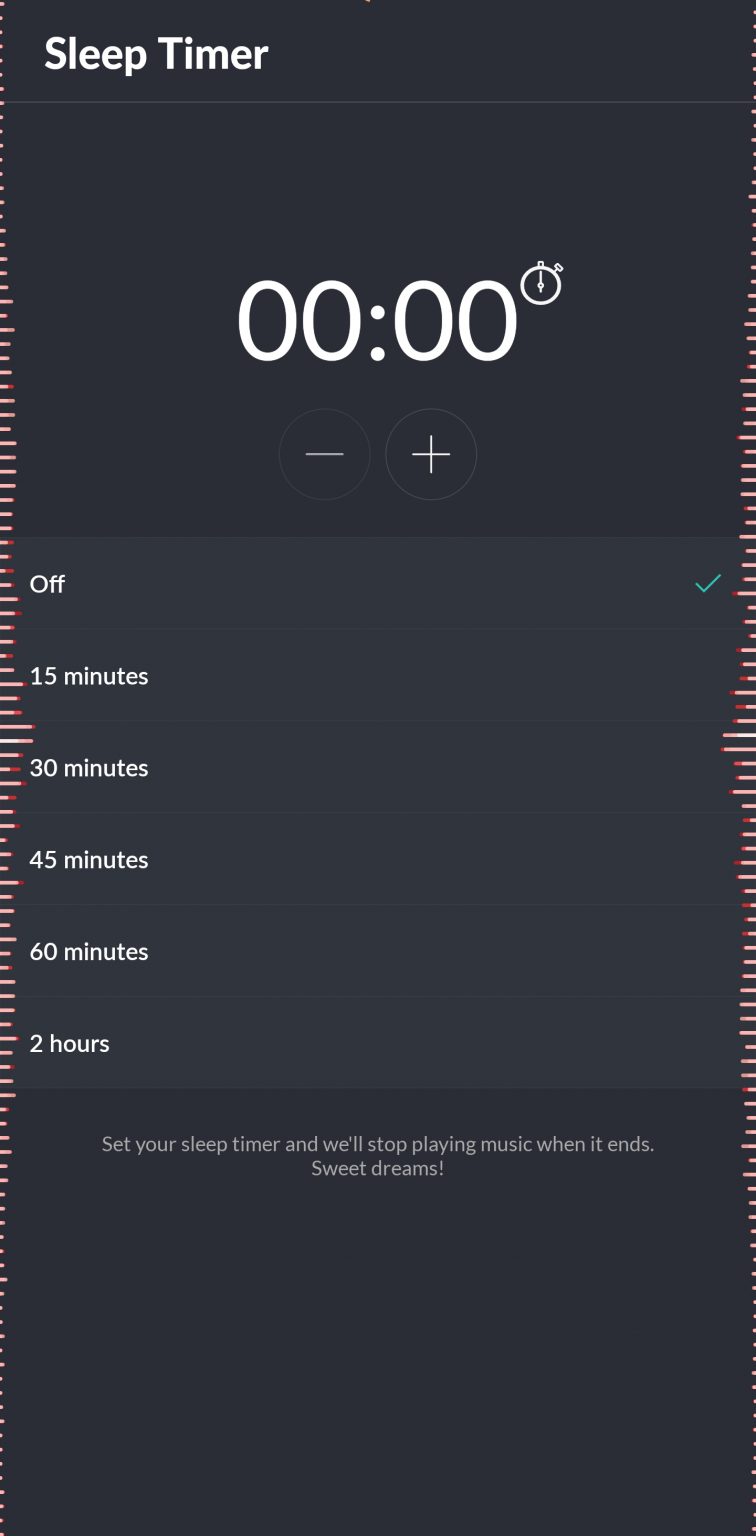The image displays a sleep timer interface, likely from a smartphone application designed for managing audio playback duration. The background is predominantly gray with subtle, short red lines running vertically along the sides. At the top-center, the text "Sleep Timer" is written in white. Below this, there are four zeros with a small animated icon of a stopwatch and a bell, also in white. On either side of the numeric display, there are plus and minus buttons to adjust the timer.

The timer options are presented in a vertical list format, featuring the following durations: "Off" with a green check mark next to it, 15 minutes, 30 minutes, 45 minutes, 60 minutes, and 2 hours. Each duration appears selectable based on the interface design.

At the bottom, a white text message reads, "Set your sleep timer and we'll stop playing music when it ends. Sweet dreams." The overall design and functionality suggest that this interface belongs to a mobile app that allows users to listen to music or audio while setting a timer to automatically stop playback after a certain period, ideal for use before or during sleep.